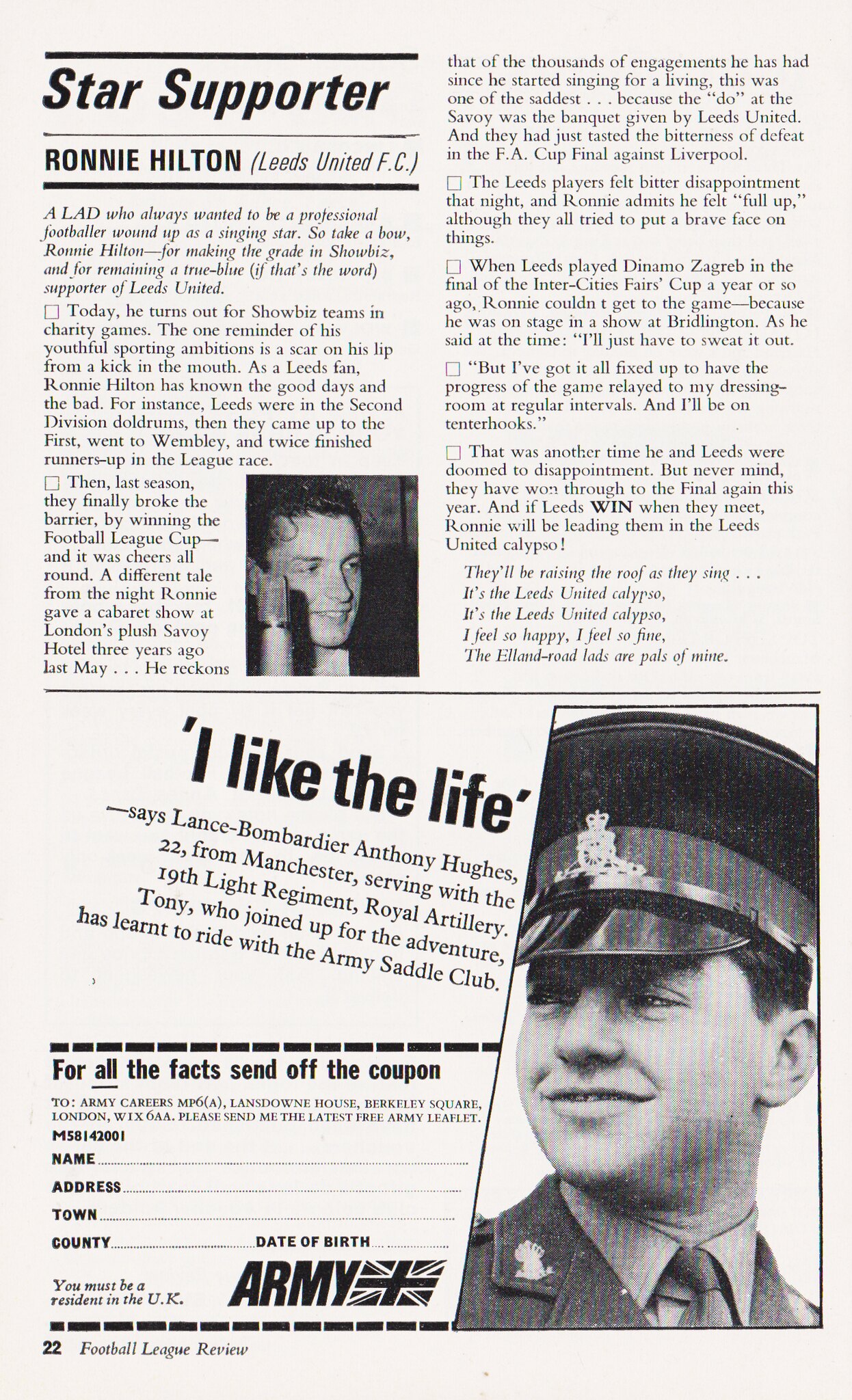This vertical, black-and-white newspaper clipping features two distinct sections. At the top, it proudly presents star supporter Ronnie Hilton of Leeds United FC, including a small black-and-white photograph of Hilton, showing him looking away from the camera. The accompanying article delves into his support for the soccer team, ending with a cheerful poem: "They'll be raising the roof as they sing. It's the Leeds United Calypso. It's the Leeds United Calypso. I feel so happy. I feel so fine. The Eland Road lads are pals of mine." 

Beneath the article lies an advertisement for the British Army. It showcases a black-and-white photo of Lance Bombardier Anthony Hughes, a 22-year-old soldier from Manchester serving with the 19th Light Regiment Royal Artillery, wearing a military hat. The ad quotes Hughes: "I like life," and notes that he joined the army for adventure and has learned to ride with the Army Saddle Club. A recruitment coupon at the bottom encourages readers to fill in their details and mail it for more information, accompanied by the British flag. The bottom left corner of the page marks it as number 22, identified as part of the Football League Review publication.